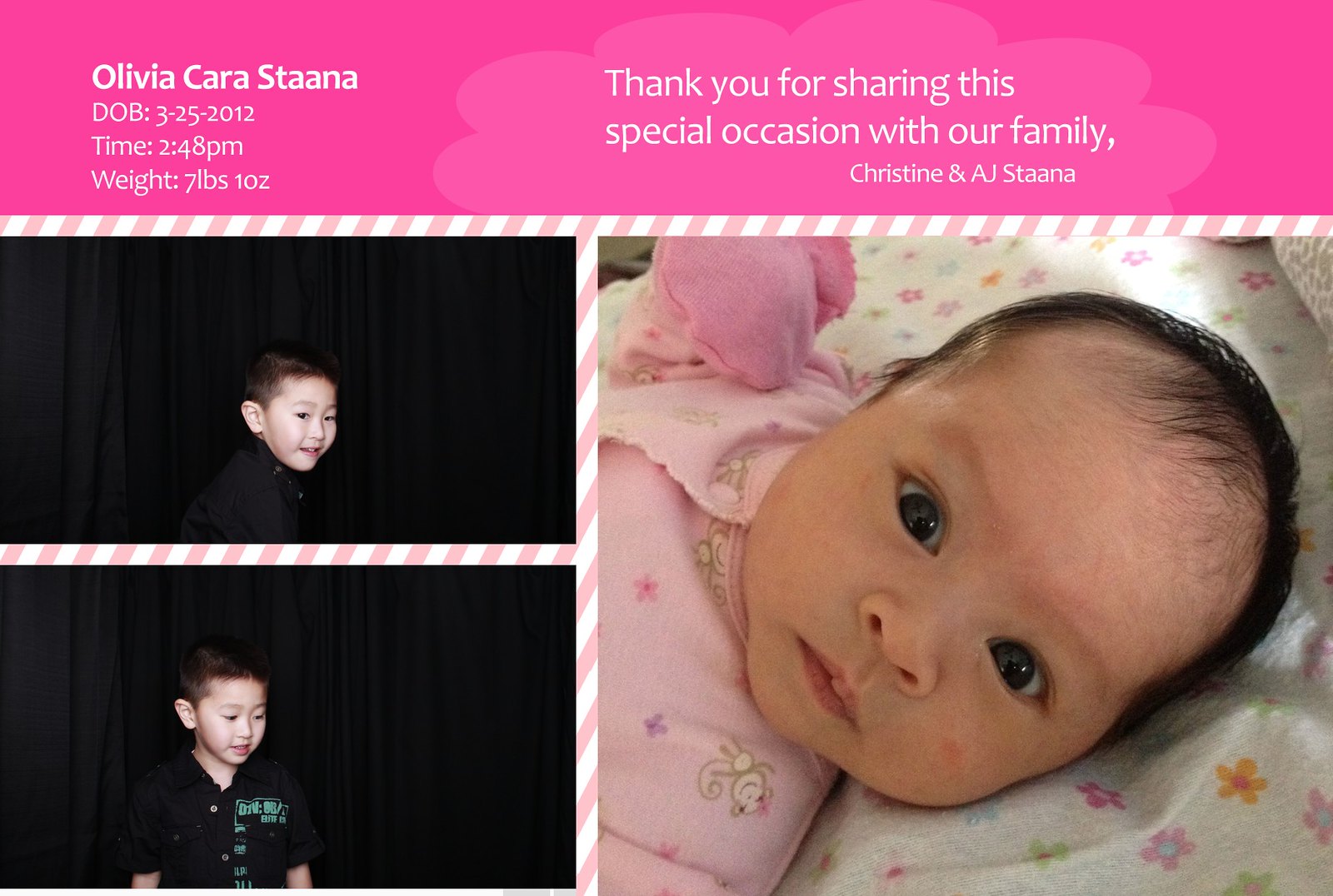The image is a beautifully crafted birth announcement or thank you card for a special occasion, celebrating the arrival of a baby girl named Olivia Cara Stana. The card is rectangular, with a prominent pink stripe or rectangle at the top, adorned with a lighter pink cloud-like background. In a delicate white font, it reads: "Olivia Cara Stana, date of birth: March 25, 2012, time: 2:48 PM, weight: 7 pounds, 10 ounces." Beneath this, there is a heartfelt message: "Thank you for sharing this special occasion with our family, Christine and A.J. Stana."

The card features three photographs divided by white and pink diagonally striped borders. On the far right, there is a lovely photo of newborn Olivia, cleaned up and dressed in pink pajamas, lying on a white blanket, wide-eyed with black hair and dark brown eyes. The central part of the card is dominated by her image.

On the left side of the card, there are two stacked photographs of Olivia's older brother, approximately three to four years old. He is depicted wearing a black shirt with green print, looking downward and smiling in one photo, and gazing straight ahead or to his right in the other. The background of these photos appears to be a sheet featuring gold, red, and blue stars, adding to the festive and joyous atmosphere of the announcement. The card captures the tender moments of welcoming a new family member and cherishing sibling togetherness.